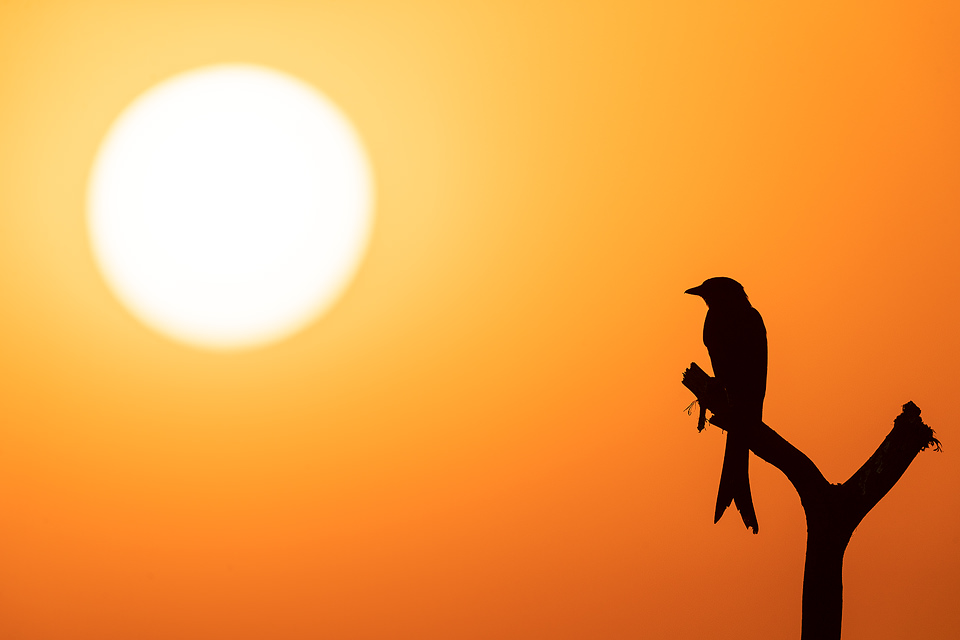The photograph captures a striking scene of a bird perched on the left edge of a gnarled, Y-shaped branch, both in black silhouette against an evening sky ablaze with shades of orange and yellow. The sky darkens around the edges and brightens towards a diffused, bright white sun in the upper left corner, piercing through a haze, giving the effect of a sandstorm. The medium-sized bird, facing left with a forked tail, appears poised as if ready for swift flight. The intricate balance of the stark silhouettes against the vibrant, fiery backdrop creates a dramatic and captivating visual contrast.